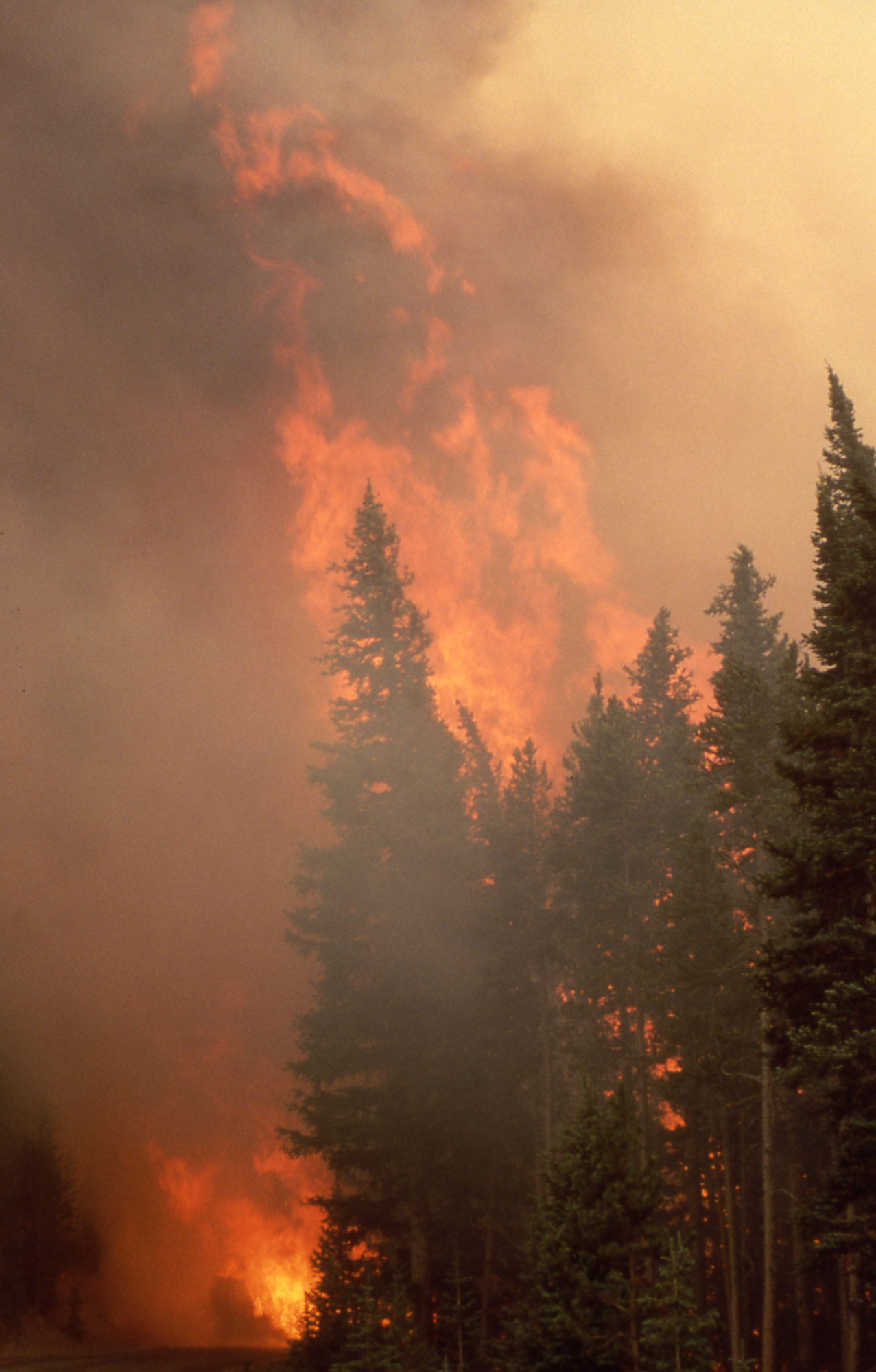In this dramatic photograph of a forest fire, taken during midday, we are observing the scene in portrait mode. The focal point is a row of tall, pointed conifer trees, likely pine or fir, standing on the edge of the forest, situated on the bottom right quarter of the image, rising around 10-20 stories high. Their branches are visible before the canopy starts, and these trees are still green, not yet caught in the blaze. 

Behind this line of trees, a ferocious inferno rages with towering flames in deep orange, red, and yellow hues that soar well above the treetops. The fire is so intense that it obscures any potential background details. Greyish-brown and black smoke billows upwards, filling the sky and forming thick, dark clouds especially noticeable in the upper corners of the image. 

The sheer scale of the fire and the dense smoke give a sense of impending doom as the fire appears to be spreading, with smaller orange flames licking up from the bottom left center of the photograph. Despite the trees in the foreground remaining seemingly untouched, the advancing blaze frames an alarming scene of natural devastation.